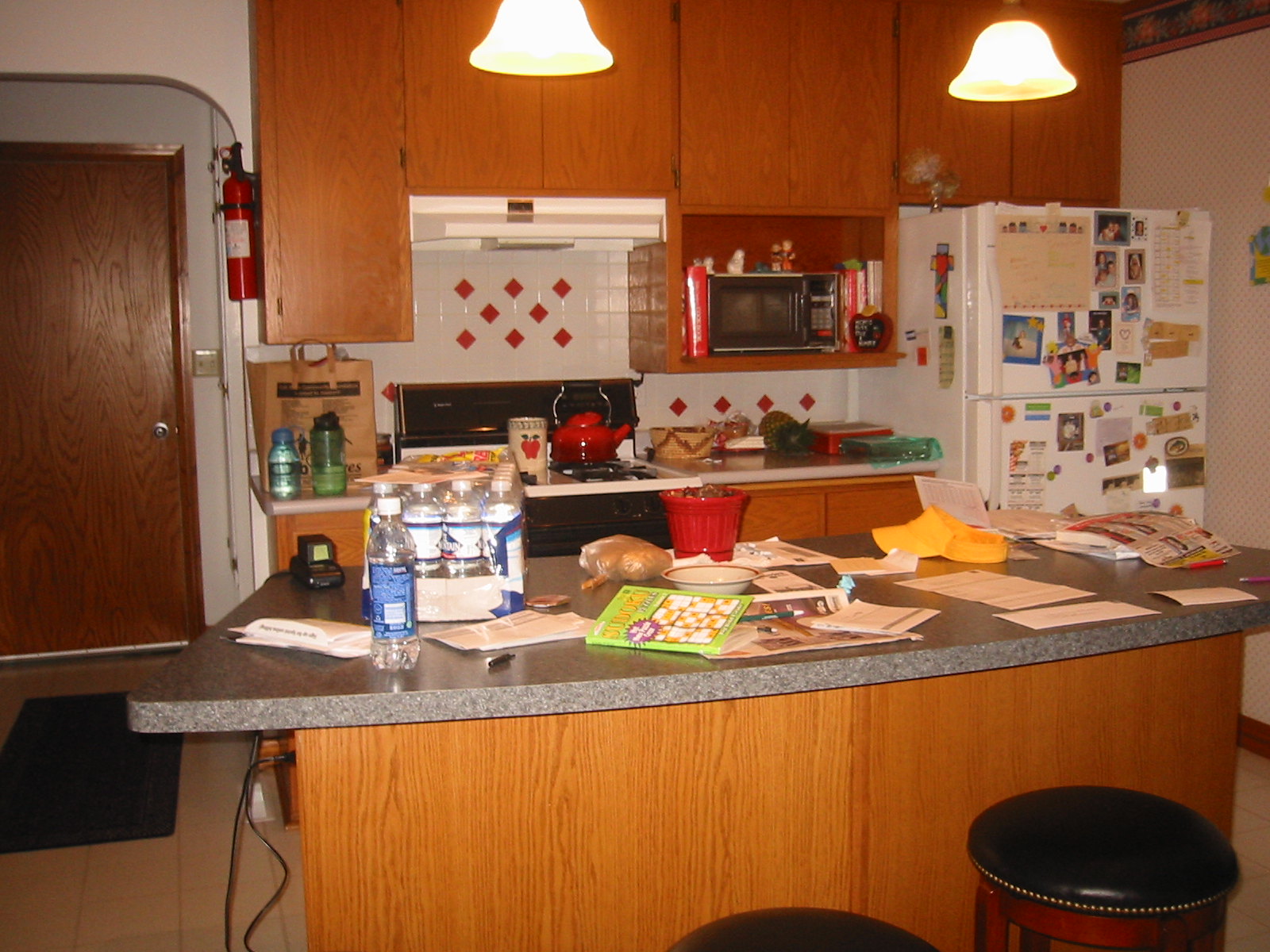In this detailed photograph, we observe a cozy, well-lived-in kitchen, or possibly a walk-in kitchen, with an island taking center stage. The island features a tall kitchen counter, and in the bottom right-hand corner, two wood-based, cushioned barstool seats are visible. These seats are upholstered with a black soft material adorned with decorative yellow dot lines. 

On the kitchen counter, there is a case of water, with a single bottle positioned to the left. The center of the island bears a variety of items, including a crossword puzzle book, a cereal bowl, newspapers, and scraps of paper. To the right, additional papers such as bills, envelopes, and what appear to be coupons are scattered.

The top right-hand side of the photo showcases a white refrigerator, festooned with pictures of children and an array of magnets on both the freezer and refrigerator doors. Adjacent to the fridge, nestled in a cubby space, is a compact microwave. Further to the left, a stovetop oven is visible, with a dark red and light red kettle resting on one of its burners. Nearby, bottles of water are stored. 

Above the scene, two large, bright wall lights illuminate the kitchen area. On the far left side of the room, a door leading outside is visible, with a red fire extinguisher mounted on the wall next to it, ensuring safety within this welcoming kitchen space.